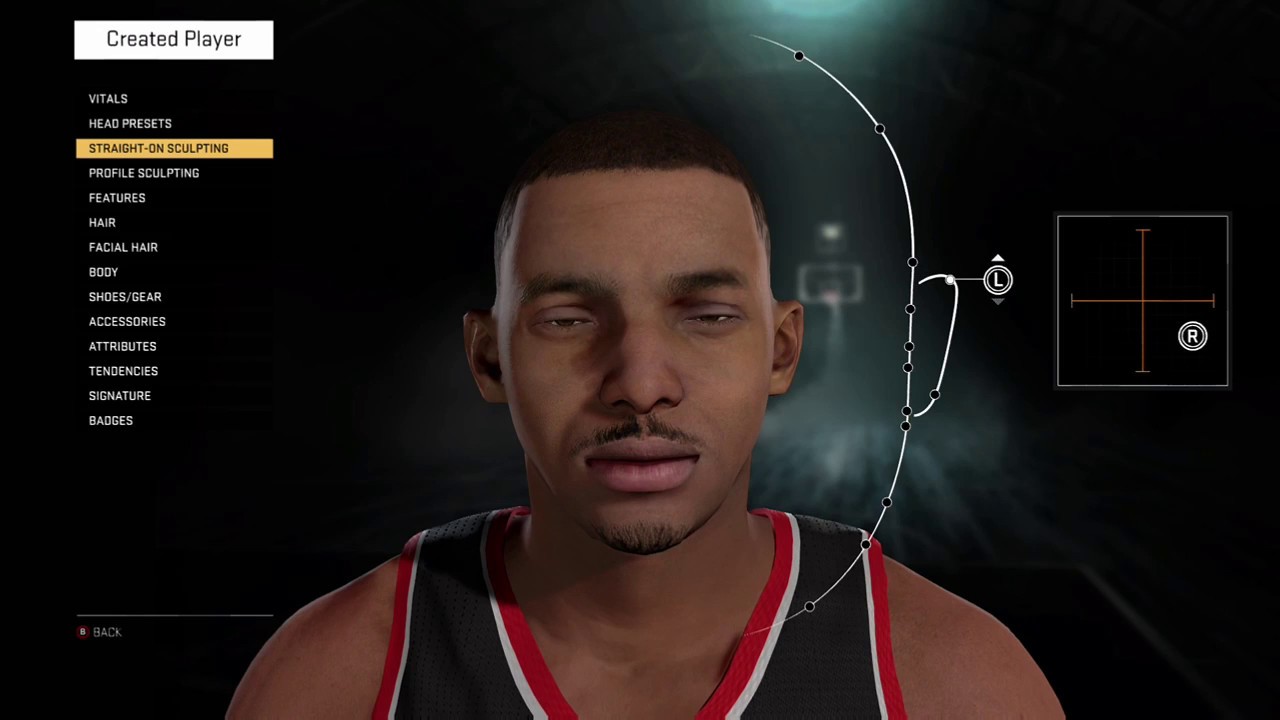The image depicts a web page interface designed for creating avatars, featuring a predominantly black background. At its center, there is a highly realistic, computer-generated representation of a man. The avatar is of a black man with medium brown skin, sporting a mustache and goatee. He is dressed in a dark gray, sleeveless sports jersey, resembling a basketball jersey. The jersey is accented with red and white borders around the neckline and armholes, suggesting attention to design detail.

On the right side of the avatar, there is a semi-circular icon, appearing to be a tool or device marker, possibly for editing or customizing the avatar's features. In the upper left corner of the interface, a white rectangle with gray text reads "Created Players." 

Beneath this heading, a list of customization categories is displayed in white text against the black background. The list includes "Vitals," "Head Presets" (which is highlighted in a yellow rectangle indicating it's selected), "Sculpting" in a black font, followed by "Profile," "Shape," "Sculpting," "Features," "Hair," "Facial Hair," "Body," "Shoes/Gear," "Accessories," "Attributes," "Tendencies," "Signature," and "Badges."